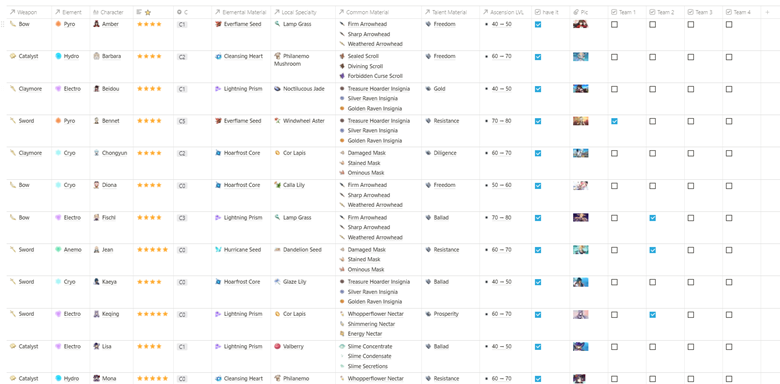This image showcases a meticulously detailed table designed to organize and store information, likely related to a video game or another type of gaming activity. The table consists of a white background with rows and columns separated by thin gray lines. The header row features a light gray background, with each entry—except for a series of checkboxes at the end—beginning with an arrow pointing to the upper right.

The columns, from left to right, are labeled as follows: Weapon, Experts, My Character, a Star icon with a gray outline, a Setting logo marked with the letter C, External Material, Local Specialty, Common Material, Talent Material, Ascension Level, followed by checkbox columns labeled as Habits, Pick, Team 1, Team 2, Team 3, and Team 4.

Every row in this table contains specific information under these categories, and most entries feature a small thumbnail icon that visually represents the text. For example, the first cell under the "Weapon" column displays the word "Bow" along with an image of a bow, while the subsequent cell under "Weapon" in the second row shows "Catapults" paired with an image resembling a catapult projectile.

In total, the table comprises 12 rows. The checkboxes in the team sections indicate team selections, filled with a blue background and white checkmarks. Notably, the fourth entry features the weapon "Sword" with the element "Pyro," marked as part of Team 1. Team 2 includes the seventh and eighth entries, labeled as "Bow" and "Sword" weapons, respectively, and the tenth entry, which lists "Sword" and the element "Electro."

The table also lists various elemental types such as Pyro, Hydro, Electro, Cryo, and Anemo, each depicted with its own distinct color symbol. For "Common Materials," each character or class has three different materials specified. The remaining categories typically contain a single entry per character or class.

The detailed and structured layout of this table allows for easy tracking and management of game-related data, providing comprehensive insights into each character or class’s attributes and team assignments.